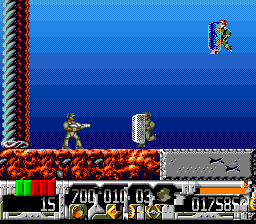This image is a detailed freeze-frame from a video game. The predominant background is blue, with a vertical pattern of red and gray running down the left side. In the center, there are two characters standing on a main stage. One character is striking a distinctive kung-fu pose, with his right arm drawn back to his chest and his left arm extended forward. His legs are flexed in a sideways stance to the right. Positioned nearby is an object resembling a water heater, though its exact nature is unclear.

In the upper right-hand corner of the image, there is an undefined object descending towards the characters. The characters are standing on a red surface, possibly depicting an underground scene. Below this red layer is a metallic gray segment, which then transitions to an area filled with a variety of colors including reds, greens, grays, browns, and even coral hues, suggesting some form of intricate, possibly organic element.